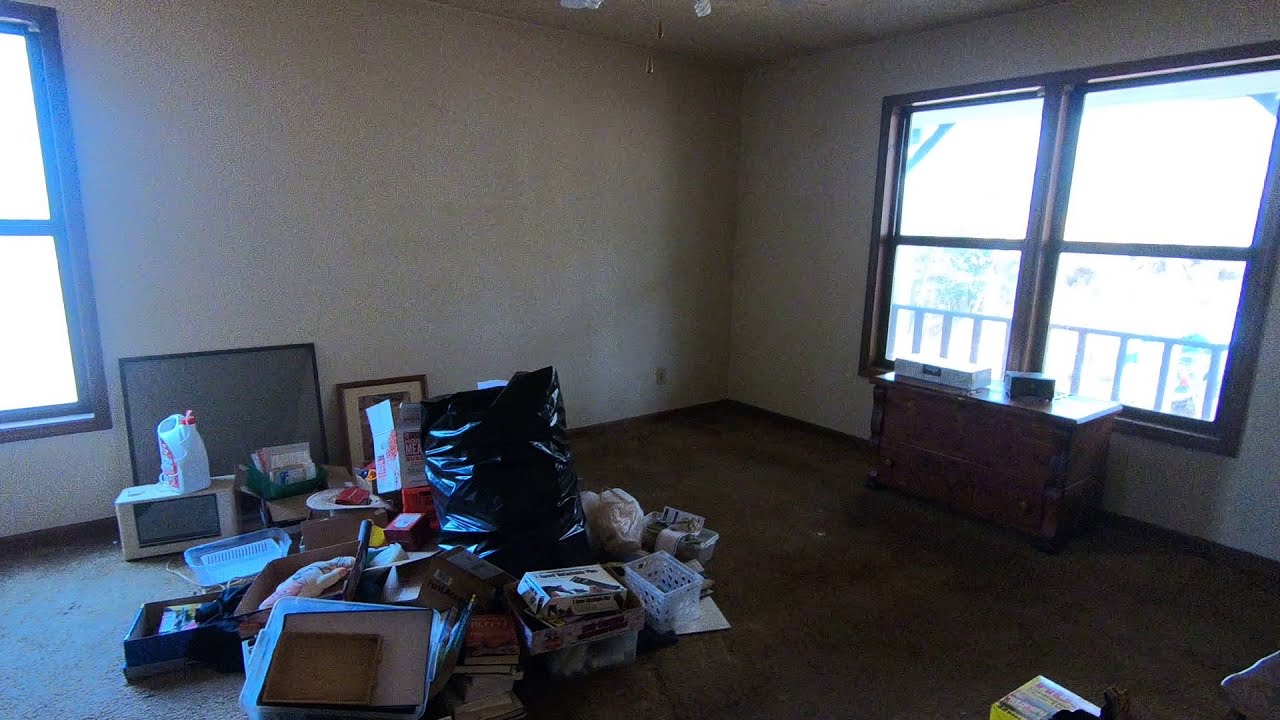The photograph captures the inside of a sparsely furnished room in a house, suggesting it's in the process of being packed up or cleaned out. Central to the image is a large pile of assorted items, including a prominent black trash bag standing upright, storage bins, cardboard boxes, an unplugged microwave, and various plastic containers. Also featured are several framed photographs that are not hung but instead leaning against the wall. The room's walls and ceiling are brown, while the carpet varies in shade from an off-white near the left to a darker brown towards the center and right.

To the right, there is a window above a wooden bureau or dresser, on top of which sits an electronic device, possibly a DVD player. Additionally, there appears to be another window towards the top left corner, allowing sunlight to stream in and subtly illuminate the otherwise cluttered space. Hanging from the ceiling, there's a fan or light fixture with dangling pull chains. The overall scene depicts a room filled with various items and trash, juxtaposed against the background of an empty, clearing-out space.